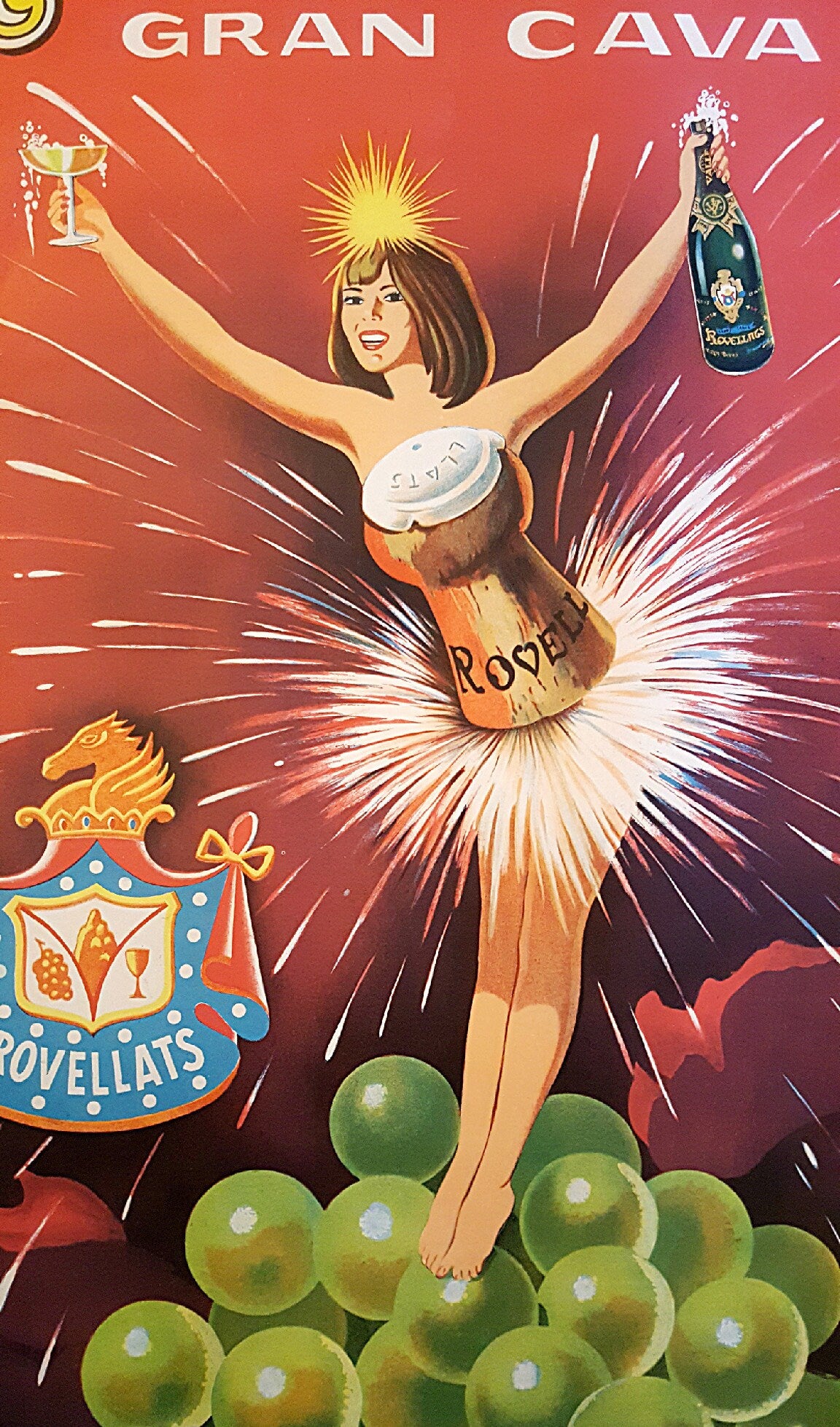The image is a promotional poster with a vibrant red background featuring white lettering at the top that reads "Gran Cava." Dominating the scene is a graphic, cartoon-style depiction of a young white woman whose torso is creatively obscured by what looks like the cork of a champagne bottle, complete with white sparks flaring out like fireworks from the bottom of the cork. The cork stretches from her knees to her neck, lending her a whimsical, almost magical appearance. She has her arms raised in a celebratory V-shape, holding a glass of champagne triumphantly in her right hand and a green bottle of champagne, bubbling over, in her left. Her head is adorned with what appears to be golden sparkles, reminiscent of sunshine.

This dynamic figure seems to be hovering or jumping above an array of grapes in green and red hues at the bottom of the poster. Directly below her is a royal blue shield crest featuring a winged horse and inscribed with the word "Provetellus" or a similar variation. The entire scene is visually striking and playful, capturing the effervescent joy associated with champagne.